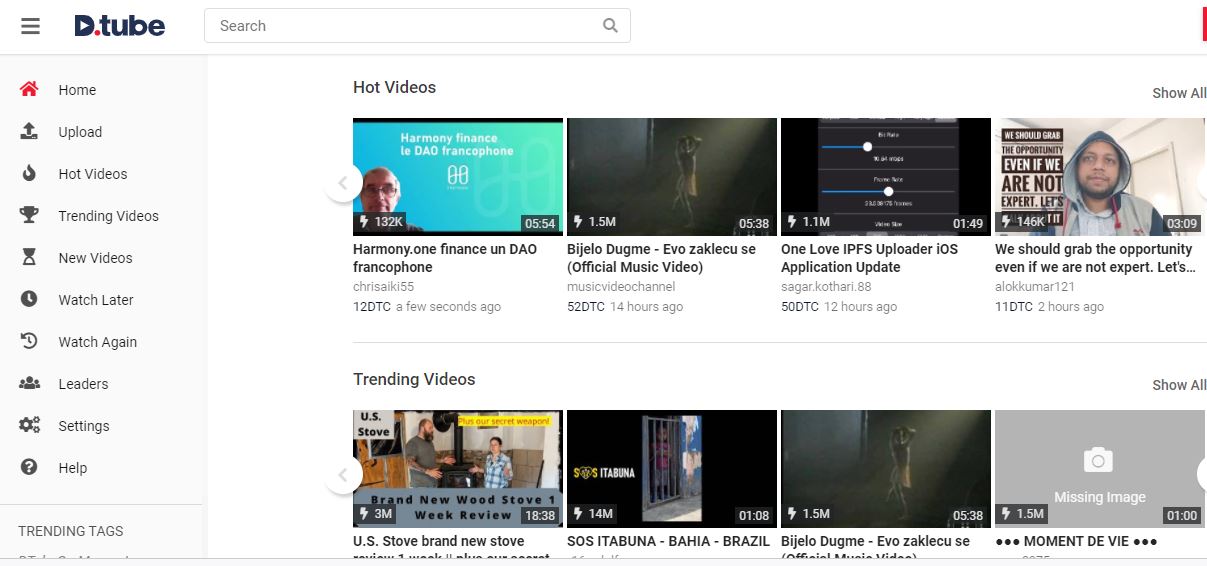This image depicts a screenshot of the website .tube. The webpage features a clean, white background and a three-line, hamburger menu icon positioned in the top left corner. Next to the menu icon is the .tube logo, with "T-U-B-E" written in bold blue text accompanied by a play button symbol.

Below the logo, a prominent search bar allows users to quickly find content. The left quarter of the page displays a vertical navigation menu with several options: Home, Upload, Hot Videos, Trending Videos, New Videos, Watch Later, Watch Again, Leaders, Settings, and Help. At the bottom of this menu, there is a separate section labeled "Trending Tags." Currently, the "Home" option is highlighted in red, indicating it's the active page.

The right three-quarters of the page are dedicated to featured video content. At the top-right corner, a "Show All" link is available for the "Hot Videos" section. Under the "Hot Videos" heading, four video thumbnails are displayed, arranged horizontally. Below this section, another set of four video thumbnails is labeled "Trending Videos." However, the fourth thumbnail in the "Trending Videos" row displays a placeholder image with the text "missing image."